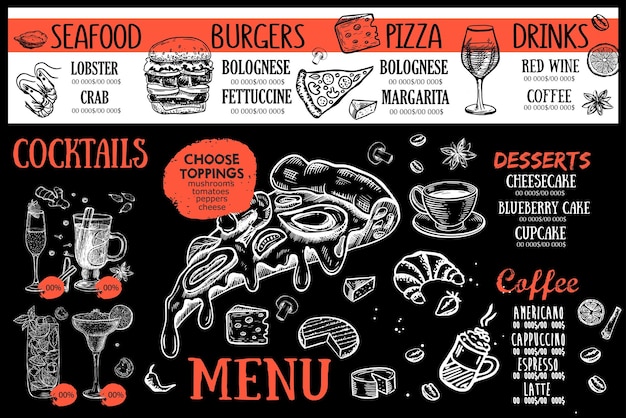This image depicts an intricately illustrated menu set against a predominantly black background with white and black accents. Dominating the top of the menu is a bold, red banner that categorizes the offerings into seafood, burgers, pizza, and drinks. Below this banner, the menu details entrées such as lobster, crab, fettuccine bolognese, and margaritas, with side notes for red wine and coffee under the drinks section.

The menu is richly decorated with clip art and illustrations. In the center, an image of gooey pizza is highlighted with a note reading "choose toppings," listing mushrooms, tomatoes, peppers, and cheese as options. The lower section on the left features different cocktails, sketched in various glass types like wine, champagne, and margarita glasses. Off to the right, there is a section for desserts and coffee, enumerating items like cheesecake, blueberry cake, and cupcake, alongside coffee options including Americano, Cappuccino, Espresso, and Latte.

Additional illustrations of food items like croissants, vegetables, and several drawn cocktails complement the text. At the very bottom of the menu, the word "MENU" is prominently written in large, red letters, tying together the overall detailed and visually engaging presentation.